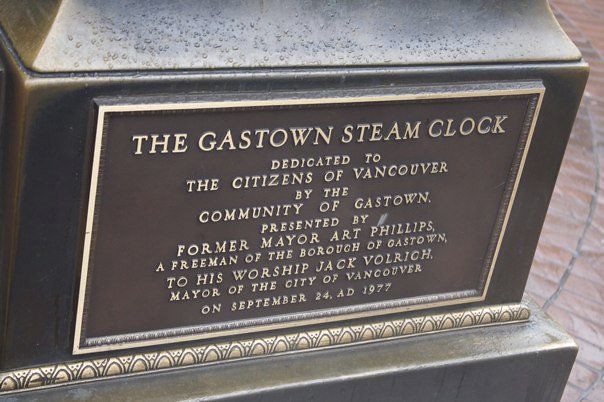The image showcases a bronze plaque at the base of the Gastown Steam Clock in Vancouver. The plaque is dedicated to the citizens of Vancouver by the community of Gastown and was presented by former Mayor Art Phillips, a Freeman of the borough of Gastown, to his worship Jack Volrich, Mayor of the City of Vancouver, on September 24, AD 1977. The plaque sits on brown cobblestones and features a rectangular, bronze background with gold-colored print and a gold border. Below the main inscription, there is a golden stripe adorned with half-circular designs. The scene appears to be wet, with water droplets visible on the plaque and the adjacent pathway.